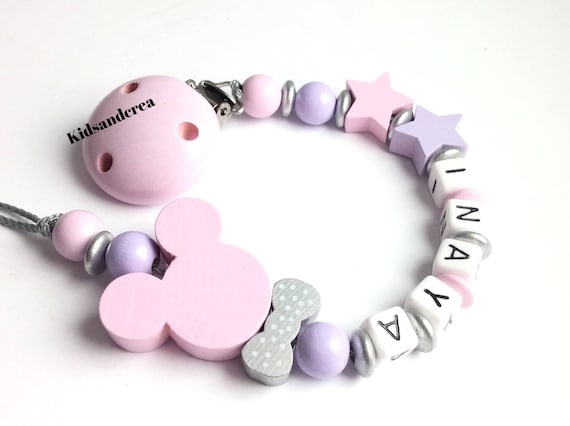This image features a child's bracelet belonging to a little girl named Anaya. The bracelet, resembling a friendship bracelet, is set against a white background, curled in a U shape. It is primarily pink and purple, adorned with pastel-colored beads and charms. Among these charms is a noteworthy pink bead shaped like Mickey Mouse's head, and a charming gray bow with white polka dots. There are small white square beads with black letters spelling out "Anaya," separated by delicate silver disc-shaped beads. The bracelet strings through a pink bead at one end, attaching to a fabric hoop at the other, which functions as the clasp. The entire bracelet is strung on a gray string and sprinkled with various pink and purple beads, and star-shaped beads, giving it a delightful and playful appearance.